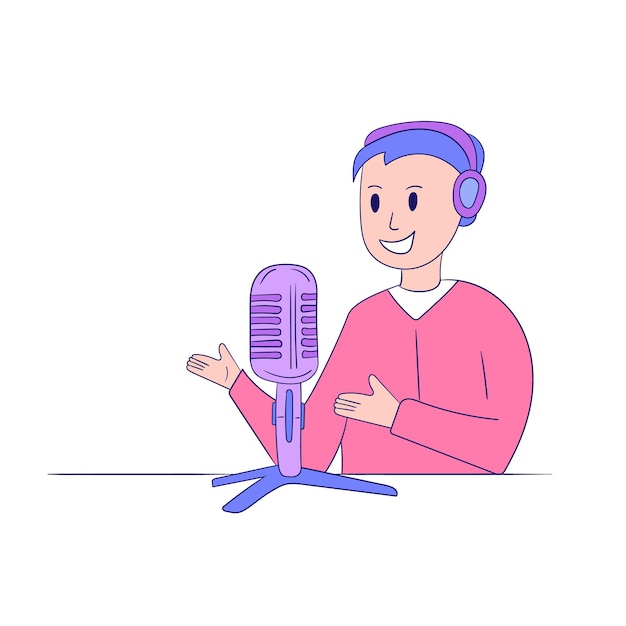This image portrays a detailed cartoon drawing set against a white background, depicting a person from the waist up with a cheerful and positive demeanor. The character has short purple hair and is wearing matching purple earphones. They have light beige skin and simple black dot eyes, suggesting a minimalist artistic style. The person is dressed in a pink v-neck sweater over a white t-shirt. Both of their arms are bent and positioned to the right side. In front of them stands a blue tripod base supporting a purple microphone, indicating that they are possibly speaking on the radio. The character's expression is smiling, enhancing the overall upbeat vibe of the scene.